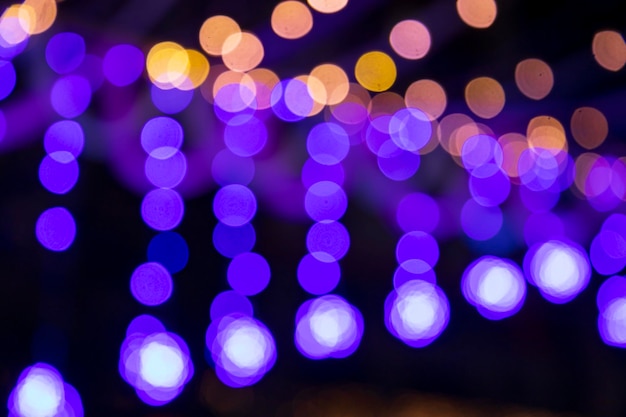The image showcases a series of bouquet-style lights on a black background, creating a vibrant and captivating visual. The lights are arranged in colorful, overlapping circles with varying densities and hues. At the bottom of the image, there is a concentration of purple lights with white centers, forming a row that runs from the bottom left upwards but stops short of the middle right. Blue circles accompany these purples towards the bottom, oriented in a vertical row that ascends towards the left. The top portion of the image features an array of orange, pink, and yellow lights, with colors described as peach, dark rose pink, light rose pink, and blush. These lighter colors increase in density towards the middle of the image, creating a more vibrant and densely populated display compared to the sparser arrangements at the bottom. Despite the soft focus and slightly blurry appearance of the lights, the overall image is brightly lit and clear, emphasizing the beautiful interplay of colors and circles against the dark background.